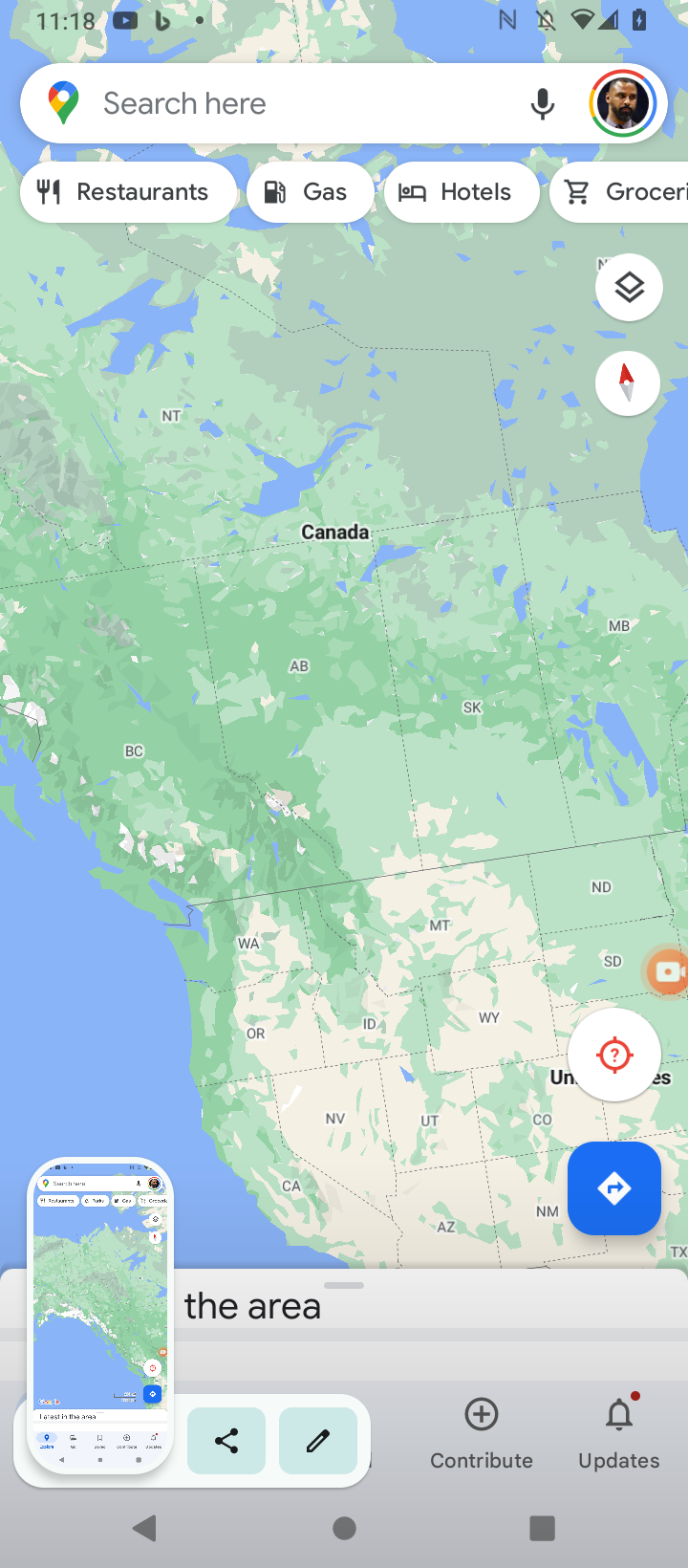The image displays a screenshot of the Google Maps app on a smartphone. The top section features the traditional white, long oval search bar with the placeholder text "Search here" in transparent gray. To the right of this bar is a microphone symbol in black and a user profile icon with a rainbow-colored border. Below the search bar, there are ovals with red text reading "Restaurant," "Gas," "Hotels," and "Groceries," though part of the word "Groceries" is cut off. The map prominently shows an aerial, computer-generated view of North America, emphasizing parts of Canada and the western and central regions of the United States. States like California, Nevada, Oregon, and Washington are clearly outlined. The map displays various topographical features, including mountain ranges, greenery, and bodies of water, with the Pacific Ocean visible to the left. The UI elements on the map suggest it is a mobile device display, with small icons like a compass, a share button, a play button, a record button, a stop button, a contribute button, and an updates icon. Additional small icons include a blue box with a 90-degree arrow, a white circle with a question mark, and an orange circle with a camera icon, located in the lower right corner of the screen.